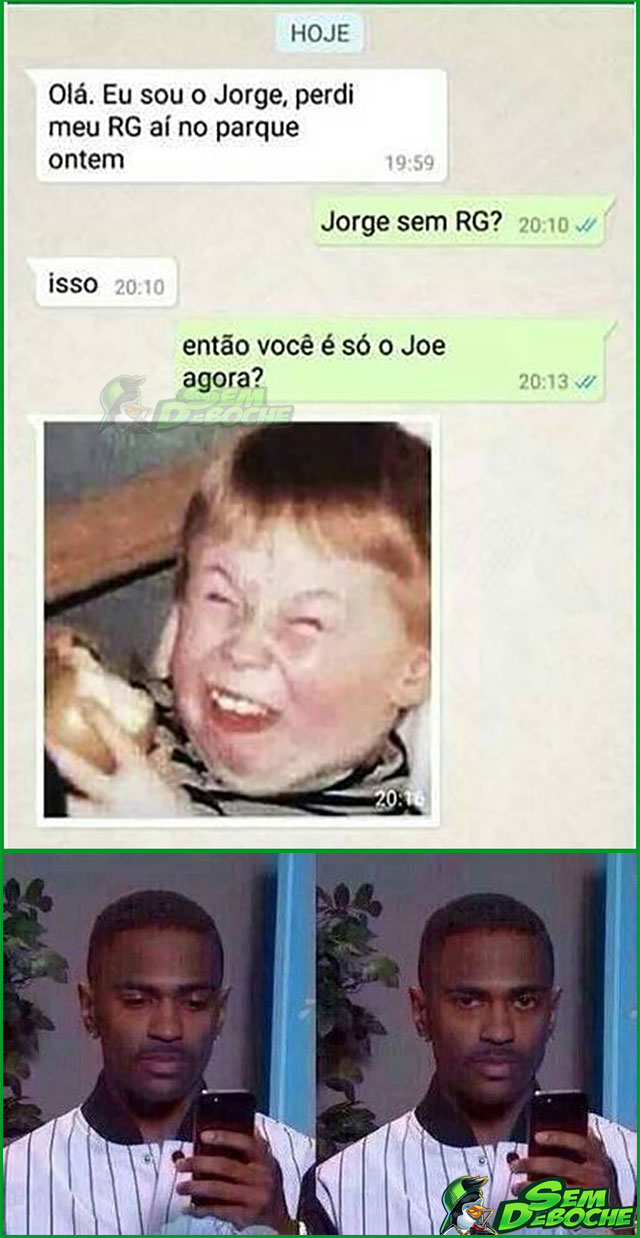The image is a screenshot of a text conversation on a phone. The background is a light beige, and the entire image is outlined with a thin green line. At the top of the screen, there is a small light blue rectangle with the name "Jorge" in it. The text messages are displayed in two different colored text bubbles: the left side features white bubbles for incoming messages, and the right side has light green bubbles for outgoing messages. 

The conversation starts with a white text bubble on the left containing the message, "Hola, eu sou a Jorge, perdi meu RG no parque ontem," which is in Portuguese and translates to "Hi, I am Jorge, I lost my ID at the park yesterday." This is followed by a light green bubble on the right saying, "Jorge sem RG?" translating to "Jorge without an ID?" The dialogue continues with a white bubble stating, "eu sou," meaning "I am," and another green bubble responding, "então você e eu sou o Jorge agora?" which translates to "so you are and I am Jorge now?"

Below the text conversation, there are three images: The first image is a medium-sized, blurry picture of a small red-haired child laughing with a mischievous expression, his eyes closed, and teeth showing. He appears to be holding an apple or a piece of bread and is wearing a black and gray shirt. The second and third images are nearly identical photos of the same black man dressed in a white and black baseball jersey. In the first photo, he is looking down at his phone, and in the second, he is looking up towards the viewer with a slight look of disdain. There is a green plant in the background and a blue wall to the right in both images. At the bottom in green text, it says, "Sim, sem RG," translating to "Yes, without an ID."

This eclectic combination suggests a playful conversation possibly mixed with meme images to add humor to the dialogue.